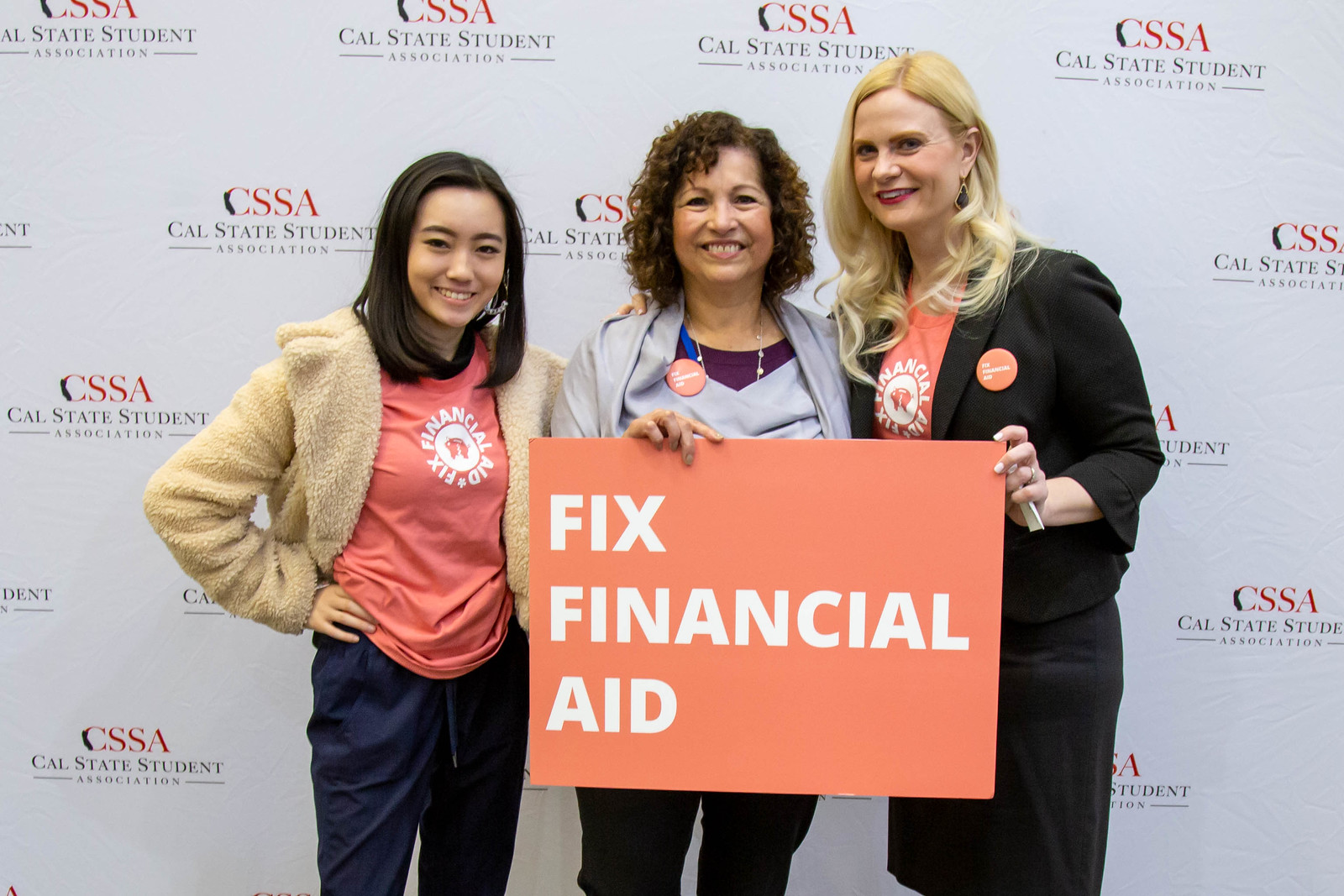Three women, standing side by side and smiling, pose in front of a photography backboard adorned with the repeated logo "CSSA" and "Cal State Student Association." Each woman holds up a sign with an orange background that prominently displays "FIXED FINANCIAL AID" in large, uppercase white letters. The woman on the left appears to be Asian, while the other two women are white. They are all dressed warmly in heavy jackets, suitable for winter weather, and the two women on the sides are wearing t-shirts featuring the "FIXED FINANCIAL AID" logo. Additionally, the two women on the right sport matching buttons, presumably advocating for the same cause. The women have distinct hairstyles: one with straight hair, one with curly hair, and one with blonde hair.